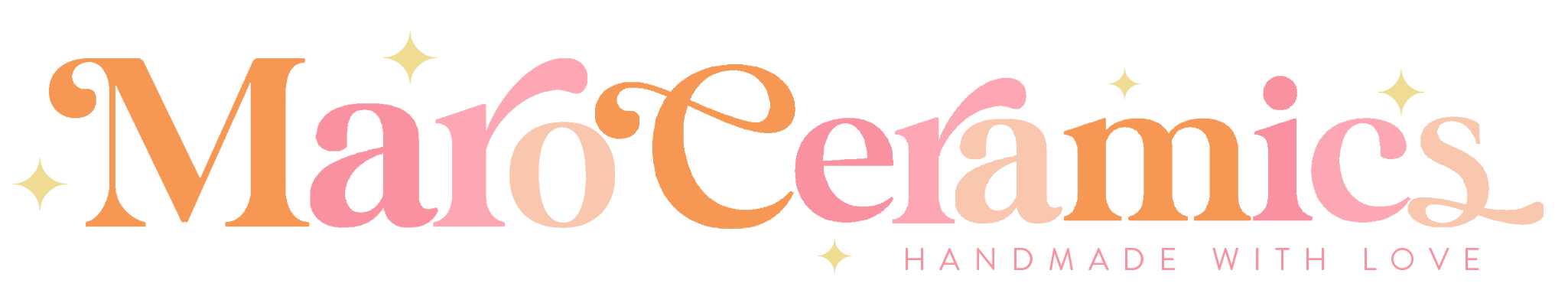The logo for Maro Ceramics is set against a white background and features a chic and playful aesthetic with artfully arranged, pastel-colored letters. The text "Maro Ceramics" is rendered in a designed font where the uppercase "M" in "Maro" is orange, followed by a pink lowercase "a" with a gold star above it, a slightly darker pink lowercase "r," and a light pink lowercase "o." The "Ceramics" portion starts with a capital orange "C," moving to a sequence of pink letters in varying shades: a dark pink "e" with a tiny star beneath it, a dark pink "r," a lighter pink "a," an orange "m" with a small star above it, a dark pink "i" with a matching pink dot, a lighter pink "c" with a gold star above, and concluding with an almost white "s."

Positioned below "Maro Ceramics" in a simple, unembellished font, it reads "Handmade with Love," adding a personal and heartfelt touch to the design. Scattered around the text are a few small, gold starbursts, enhancing the logo with a subtle celestial effect. Overall, the logo conveys an elegant yet whimsical brand image, indicative of the lovingly handmade ceramic products offered by Maro Ceramics.